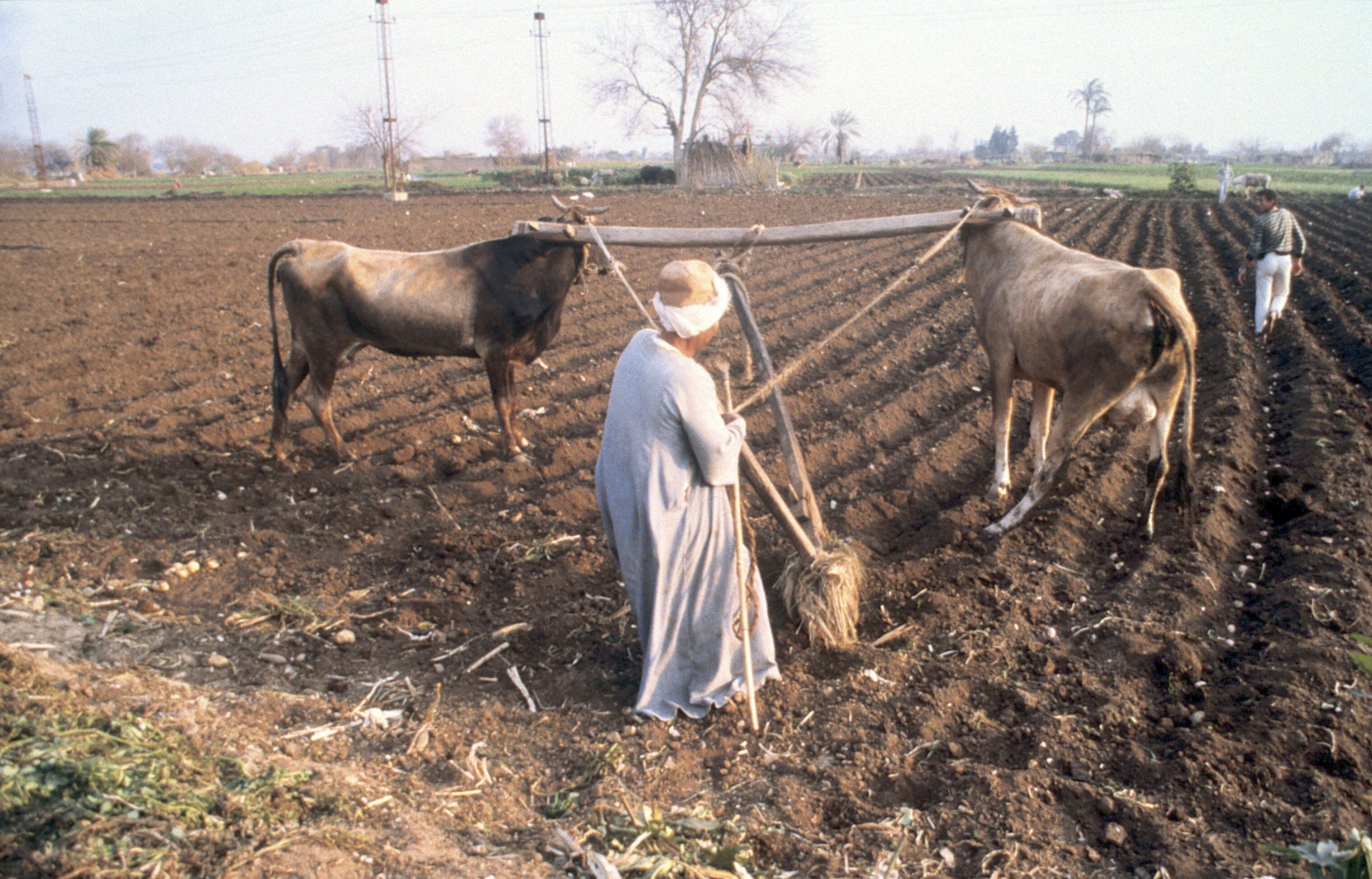In an outdoor setting that appears to be a farm, a woman is seen in the foreground, dressed in a light blue gown and a beige cap, standing behind a manually made plough tethered to the horns of two oxen. The woman holds ropes attached to this plough as she prepares to till the brown dirt field, evidenced by the freshly made ridges in the earth. Her task is set against a backdrop that blends ancient agricultural practices with modern elements, including cell towers visible in the upper left corner. Further enhancing the scene's complexity, a man walks in the background towards the far right, clad in white pants and a black-striped shirt. The field is framed with patches of green, some grass and trees peeking through on both sides, creating a vivid and timeless tableau of farm life.